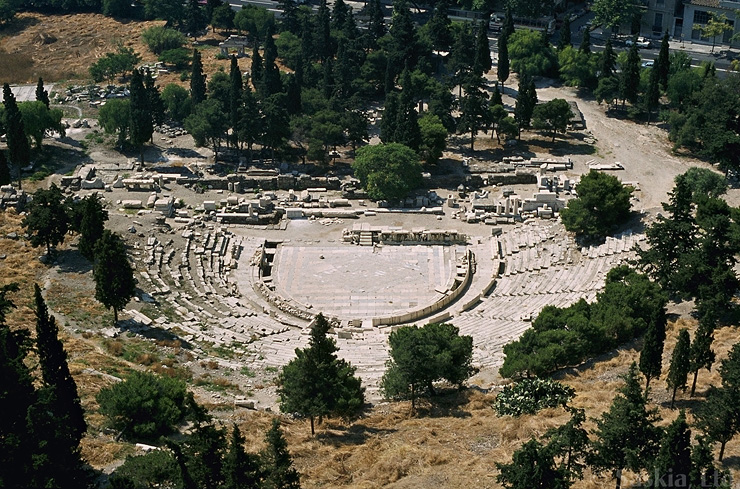This image captures an ancient amphitheater from an archaeological excavation site, positioned on a hillside. The amphitheater, shaped like a horseshoe, features a semi-circle stage in the center, surrounded by weathered brick walls and a small set of central stairs leading up to the partially ruined stage area. The amphitheater's seating is composed of white stone steps that ascend the hill; while the right side and center stairs remain mostly intact, the left side shows significant ruin. The area is strewn with rubble, rocks, and some standing pillars, indicative of the structure's ancient origins. The foreground on the hillside is dotted with sparse trees and shrubs, transitioning into tall green trees and yellowish-brown grass in the background. A dirt road runs along the right side of the image. In the distant top right, there is a street with several buildings and scattered cars, further emphasizing the amphitheater's historical contrast against modern surroundings.